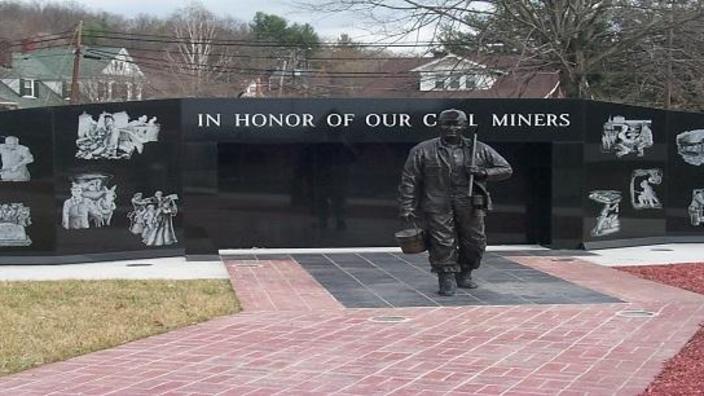This photograph is a detailed depiction of a coal miners' memorial taken in landscape mode. The centerpiece is a bronze or black statue of a coal miner, dressed in mining attire, carrying a pickaxe over his left shoulder and a bucket in his right hand. This statue stands prominently on a brick walkway that transitions from red to black bricks. Surrounding the walkway, there is a small patch of grass to the left and red mulch or gravel to the right. 

Behind the statue is a long, black stone or marble memorial wall with the inscription, "In Honor of Our Coal Miners," in white lettering. The wall features various white-etched images, possibly engraved, depicting scenes of coal miners at work spread across its expanse. The central part of the wall appears solid black, and it's suggested that a closer view might reveal additional details like names of miners.

In the background, the tops of residential houses with green and brown roofs, along with power lines, can be seen amid a landscape of trees that have either changed color or lost their leaves, indicating a fall or winter setting under a cloudy sky.